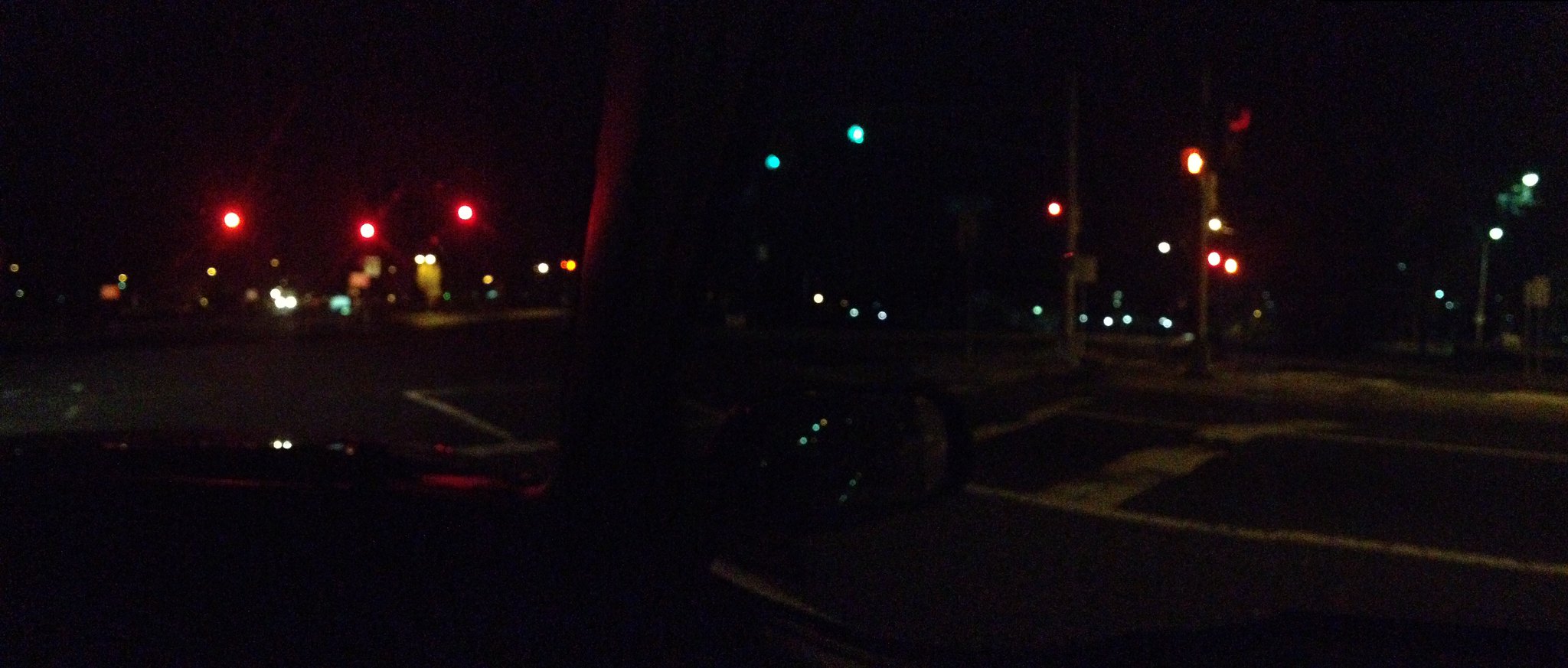A nighttime street scene captured from inside a stationary vehicle, potentially using a cellphone, camera, or dash cam. The image is predominantly dark, with details obscured by low light. Central to the composition are three illuminated red stoplights, suggesting the vehicle is stopped at an intersection. Surrounding the dark scene are various light sources from buildings, advertisements, and street lights, which dot the image with vibrant hues of red, green, orange, pink, and blue. On the right side of the frame, a white painted line, likely indicating a turn lane, can also be seen. The mix of artificial lights against the night sky creates a vivid and dynamic urban atmosphere.